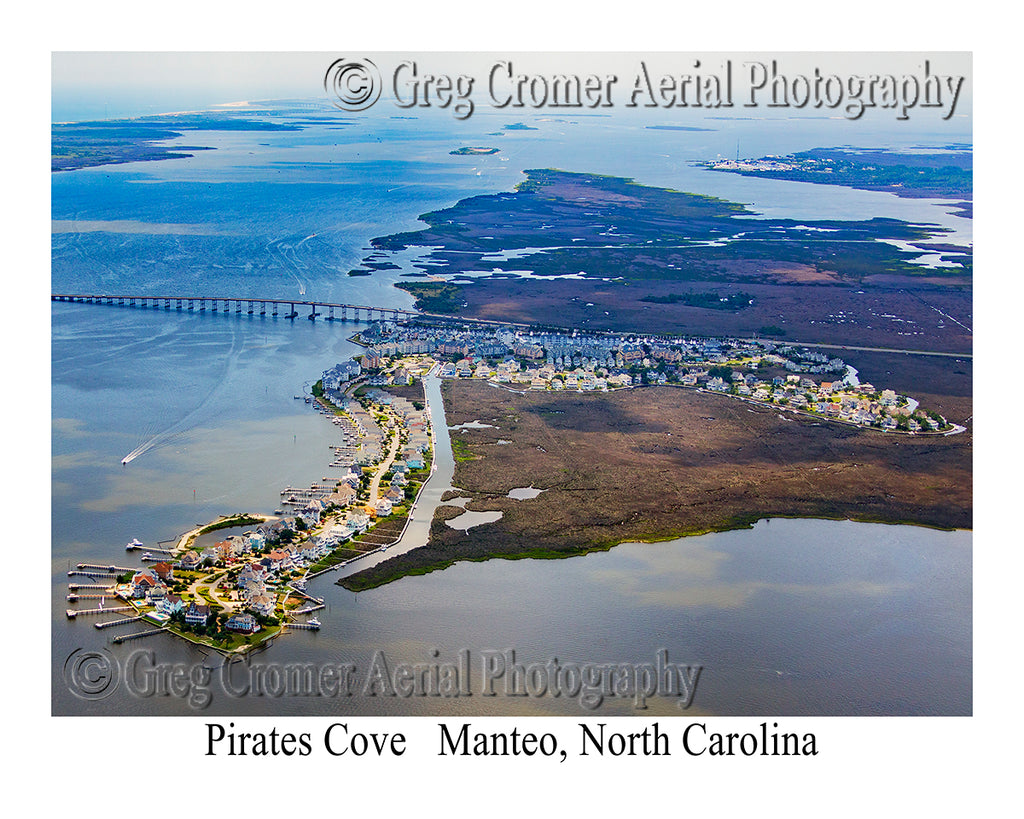This aerial photograph, taken by Greg Cromer and watermarked with "Gregor Cromer Aerial Photography" in the upper right and lower left corners, captures an intricate overview of Pirate's Cove in Manteo, North Carolina. The image prominently features a long bridge that spans across a vast body of water, appearing to be either the sea or a river, and fades out as the picture cuts off on the left side. The scene showcases several docks jutting out into the water, along with numerous buildings lining the coastline. A street is visible, leading from the dock area towards a busier section of the town, hinting at a gradual transition from a quiet coastal zone to a more bustling urban region. The landscape, primarily flat, displays patches of green amidst predominantly brown land, suggesting a mix of developed and natural terrain. In the foreground, one ship is seen approaching, with others docked further away, all under a clear, sunny sky that highlights the vivid details of this coastal area.